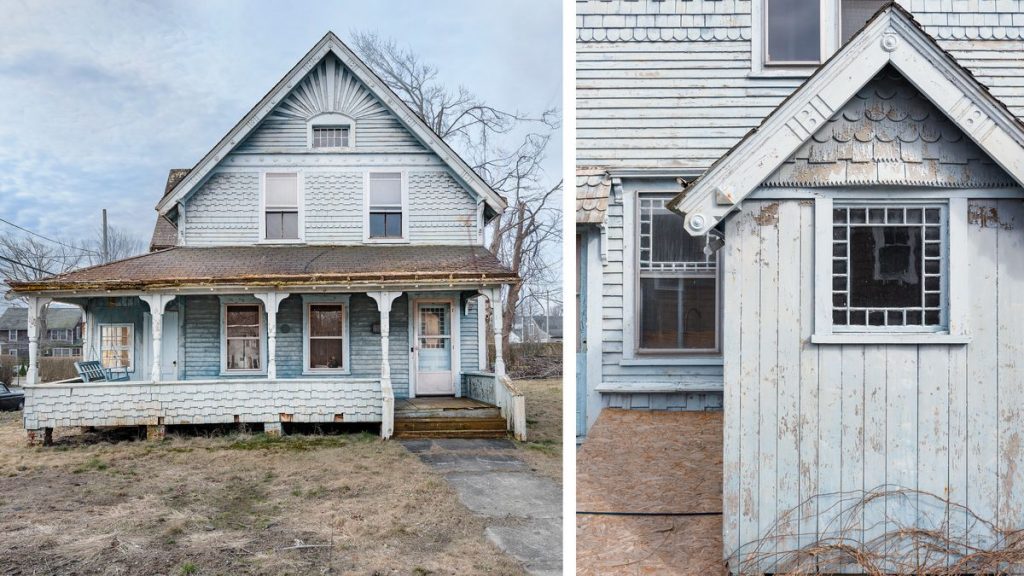The image is a split composition showcasing two perspectives of an old, worn house in need of repair, capturing both the broader context and intricate details. The left side presents a full exterior shot of the A-frame, colonial-style house marked by its faded white and light blue façade and a sloping brown roof. The house features a pitched roof that shelters a front porch, supported by aged pillars with white, covered rails, and a wooden swing hanging from the porch roof, adding to its nostalgic charm. Steps lead up to the porch, while a concrete sidewalk and patches of brown grass stretch out in front, emphasizing the unkempt, cultivated outdoor area. Surrounding the house, leafless trees enhance the rustic ambiance, alongside visible utility lines. Above, the sky is a clear blue. 

The right side of the image is a close-up, likely of the back part of the house, zooming in on the sloping roof and windows, which maintain the same white wooden paneling. This detailed view underscores the architectural elements, highlighting the textures and nuances of the house's deteriorating condition. The split image effectively juxtaposes a comprehensive and detailed visual narrative of the house's state and its architectural characteristics.